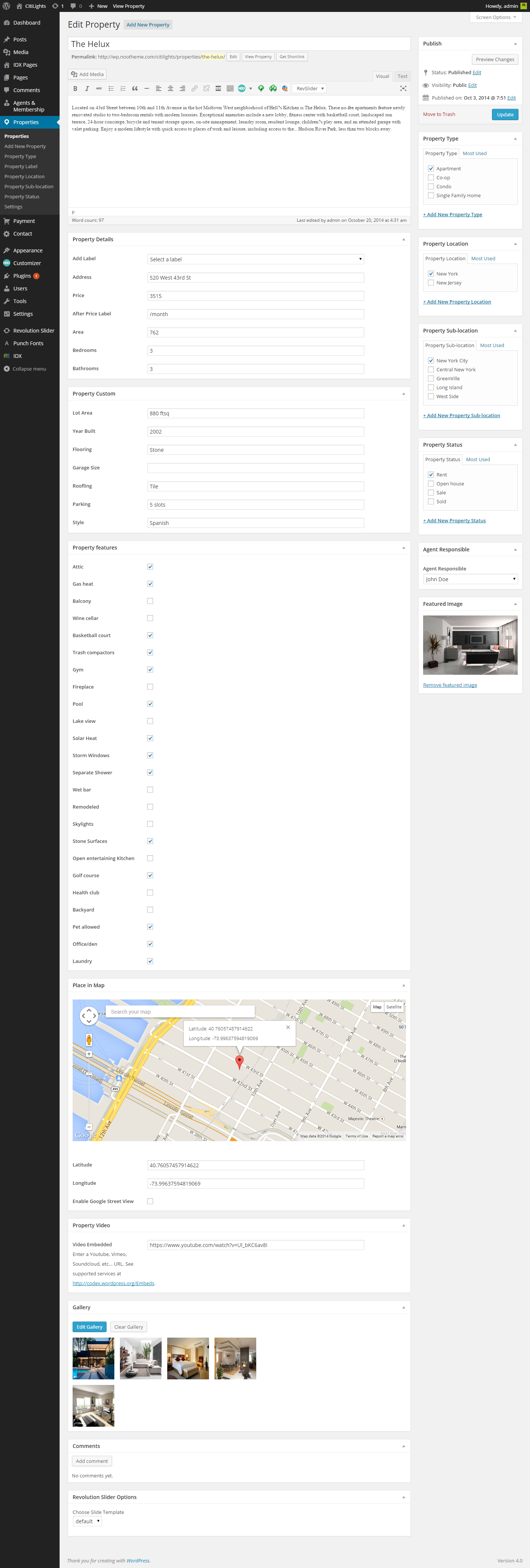A highly zoomed-out image displaying a complex interface that makes it challenging to decipher details due to the minuscule text. At the very top, black text is set against a gray background. Directly below, there is a search bar containing two words. The main body of the image features three distinct sections filled with black text.

To the right, there's an area with a blue search bar. Central to the image is a map with a small red symbol at its center. Adjacent to the map on the left, a yellow icon resembling a road appears, flanked by a blue expanse likely representing water. Scattered within this blue area are red dots, possibly indicating landmarks.

Beneath the map are five images showcasing the interiors of hotel rooms, suggesting a search for accommodation options. On the far right, five additional text-filled sections are visible. At the very bottom of the image, another search area is distinguished by an icon that appears to be a TV.